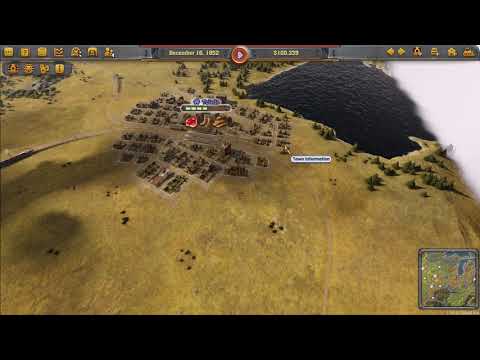The image depicts a gameplay screen from a video game set in an animated desert environment. The scene is viewed from an overhead perspective and is slightly blurry. The terrain is predominantly sandy with dark soil or terrain on the right side, accompanied by clusters of small buildings and pathways that meander through the area. The semicircular dirt path extends from the middle left to the lower center of the image. Bushes are scattered, particularly towards the upper left. In the upper right corner, there is a dark body of water with visible ripples and a white cloud above it. The top portion of the screen features a bar filled with various icons and options, possibly including a progress indicator. In the lower right corner, a square minimap provides a detailed overview of different terrains and important locations within the game world.